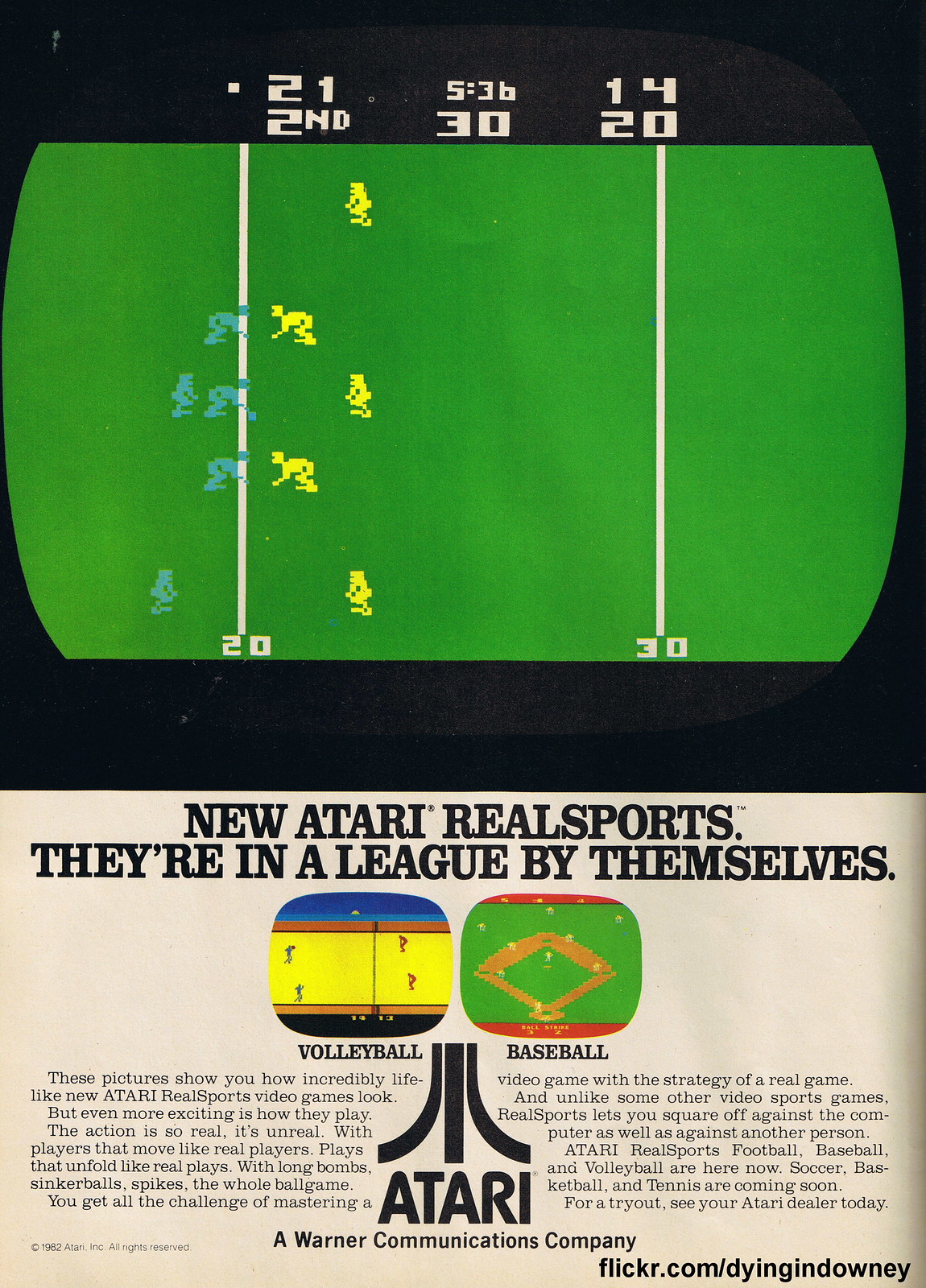This image is the back cover of a magazine from possibly the 1970s or 1980s, featuring an advertisement for the new Atari Real Sports series. The upper half of the page showcases a screenshot of an American football video game with primitive graphics typical of early Atari games. The game display shows a green field with white measurement lines, including yard markers at "20" and "30". One team, depicted in a bluish-green color, is positioned on the left, while the opposing team, in yellow, is on the right. The score is displayed as "21 to 14" in the second half, with "5:36" left on the clock.

Below the game screenshot, the ad boasts the tagline, "New Atari Real Sports. They're in a league by themselves," emphasizing the lifelike action of these new video games. Additional images highlight other Real Sports games, including volleyball and baseball, demonstrating the range of sports available in this series. The ad further includes the Atari logo, the phrase "A Warner Communications Company," and a reference to the source, "flickr.com/Dying in Downey," in the lower right corner.